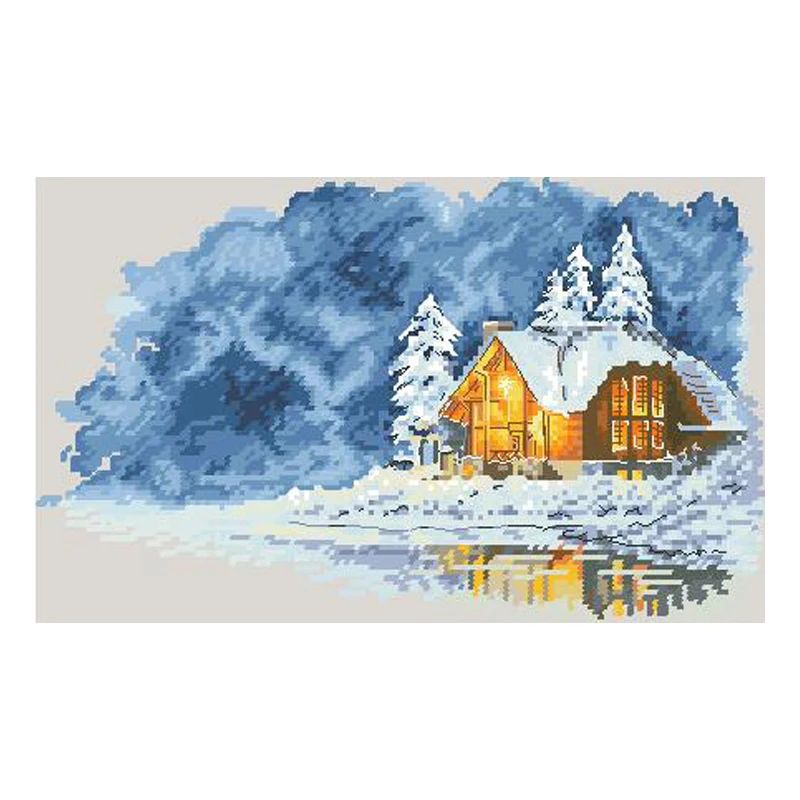This highly pixelated, computer-generated artwork portrays a cozy, well-lit two-story cabin in a wintery landscape. The cabin, offset to the right of the image, is surrounded by snow-covered evergreen trees and sits beside a reflective lake. The background features varying shades of blue, suggestive of a sky, and further accented by bluish-green and gray hues that evoke the presence of a forest. The snow-covered trees, along with the snowy roof of the cabin, clearly indicate a recent snowfall, adding to the serene and cold winter atmosphere. Despite the pixelation, the cabin's structure is discernible, displaying six windows on one visible side and a large chimney, contributing to an inviting and picturesque scene.